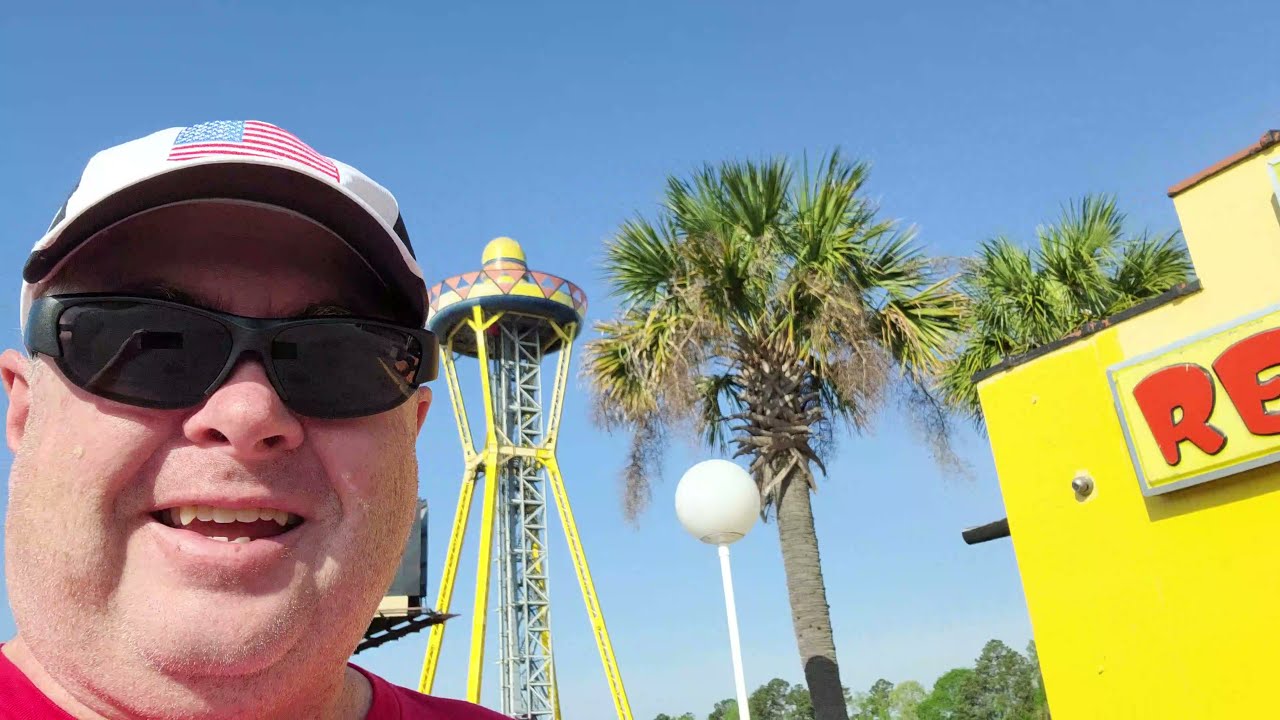The image is a vibrant outdoor scene viewed from a low angle, which emphasizes the sky as the backdrop. Dominating the center of the photograph is a tall, yellow tower with pink decorations, resembling a sombrero, hinting that the location might be South of the Border. To the right of the tower, there are two palm trees with visible green fronds and a gray trunk extending into the frame. Below these, a white, hemispherical street lamp is positioned. 

In the bottom left corner of the photograph, a man is prominently featured. He is middle-aged, slightly heavyset, and appears to be talking, with his mouth slightly open revealing his top teeth. He is wearing a red or pink t-shirt, sunglasses, and a white baseball cap featuring an American flag with a black underside on the brim.

To the far right of the image is a bright yellow building with a partially visible sign on it, showing the letters "R" and "E" in red. This building, along with the palm trees and the unique tower, contributes to a lively and colorful composition.